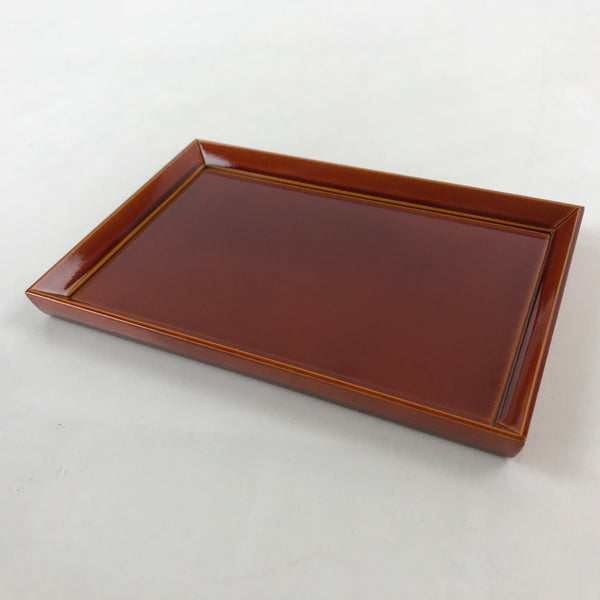This image showcases a meticulously polished rectangular tray against a grayish white background featuring subtle shadows. The tray, possibly of lacquered wood or ceramic, exudes a vintage Japanese aesthetic with its dark brown color and darker edges, standing roughly an inch tall with slightly raised edges. The light is gently reflecting off its smooth, glazed surface, particularly noticeable at the top left and bottom left corners, hinting at its well-maintained, pristine condition. The composition is simple yet elegant, with no text or additional objects present, emphasizing the craftsmanship and reflective finish of the large tray on its minimalist background.